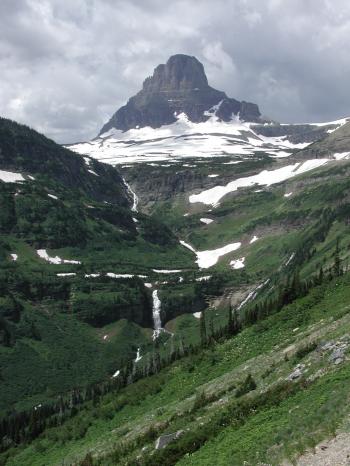This is a panoramic photo that captures a majestic alpine valley, likely somewhere in the Swiss Alps. Dominating the background is a very tall, triangular gray mountain shrouded in gray clouds, giving a moody and overcast appearance. As your eyes travel forward from the mountain's base, you encounter a mix of snow-covered areas and patches of green, indicative of interspersed meadows and sparse trees.

The landscape forms a distinctive valley, with the land on the left tilting at about a 40-degree angle to the right, mirrored by a similar slope on the right side of the image. This creates a visual play where green fields and rocky terrain blend harmoniously, occasionally revealing sporadically dispersed patches of snow. 

In the foreground, the ground slopes downward from the center-right to the bottom-left, adorned with weeds, grasses, and rocks, adding texture to the scene. The overall composition, with its diverse elements of snow-touched pastures, rocky terrain, and a towering mountain under an overcast sky, evokes the serene yet rugged beauty of high-elevation alpine environments.